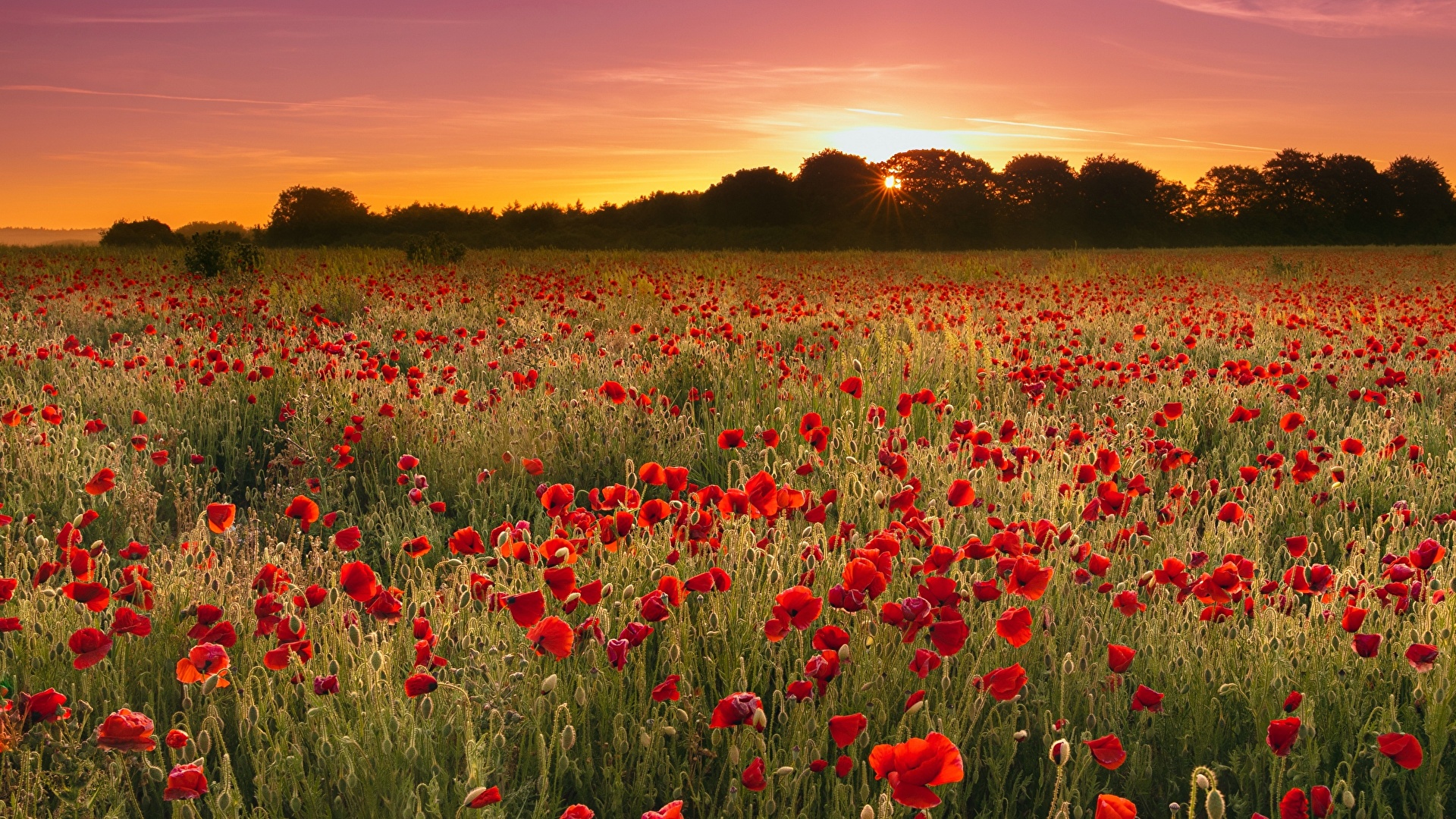The image depicts a vast and vivid field filled with primarily red flowers, possibly petunias, with dark-colored centers against a backdrop of green grass and stems. The field stretches extensively from left to right, covering much of the middle portion of the image. Buds that have yet to bloom are scattered among the flowers. In the background, there's a row of large trees partially obscuring the setting sun, which casts a radiant glow across the scene. The sky above transitions from a reddish-yellow hue near the horizon to a pinkish tint, eventually becoming purple at the very top, except around the sun where it is a bright white. The image is remarkable for its exceptional clarity and natural lighting, capturing the serene beauty of the landscape, almost resembling a computer-generated image.